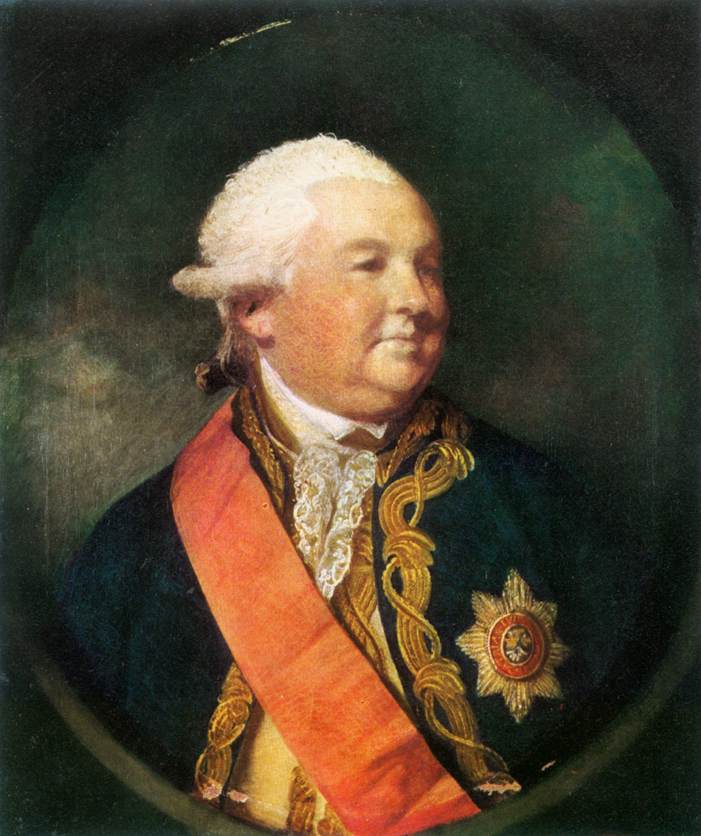This vertical rectangular oil painting portrays an elaborate portrait of an older, overweight man from the era of George Washington. He dons a prominent white wig styled with curls, tied into a low ponytail. His round, chubby face with a smug expression is looking off to the side and bears a complexion that's a mix of pale white and reddish hues. His cheeks appear somewhat tanned and crackly.

The man is adorned in a dark blue, military-type ornate jacket, featuring intricate gold braiding around the collar and edges, along with a decorative golden star on his left breast. The star has eight points, a red ring in its center, and a darker core. He is also wearing a white shirt with a fancy ruffled collar, and a red sash crosses his chest. At the bottom of the image, the edge of a cape is visible, swirling in a circular motion. The painting’s background is dark and murky, devoid of detailed elements, further emphasizing the subject's elaborate attire and distinctive features.